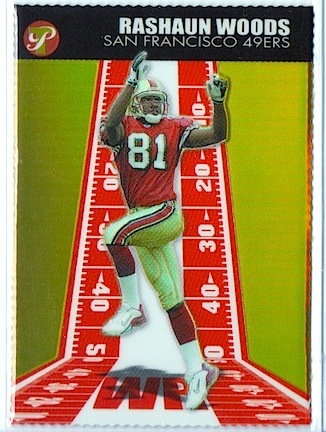The image portrays a vibrant and dynamic scene, likely from a sports card or advertisement, showcasing Rashawn Woods of the San Francisco 49ers. At the forefront is Rashawn Woods, donning a red jersey numbered 81 and white pants accented with a red stripe. He is captured in mid-action, leaping into the air with both hands raised above his head as if poised to catch a football. His left leg is bent while his right leg remains grounded, adding to the sense of movement. The football field is depicted with curved yard lines marked in red, ranging from the 10 to 50-yard lines, against a limish green background that gives a bright, colorful contrast.

At the top of the image, a thin black bar contains the player's name and team: "Rashawn Woods, San Francisco 49ers." In the top left corner, a burgundy circle with a gold-engraved "T" and a cursive "P" adds a distinctive feature, possibly a logo. The visually striking graphic design enhances the excitement and dynamism of the scene, making it a compelling and eye-catching representation of football action.